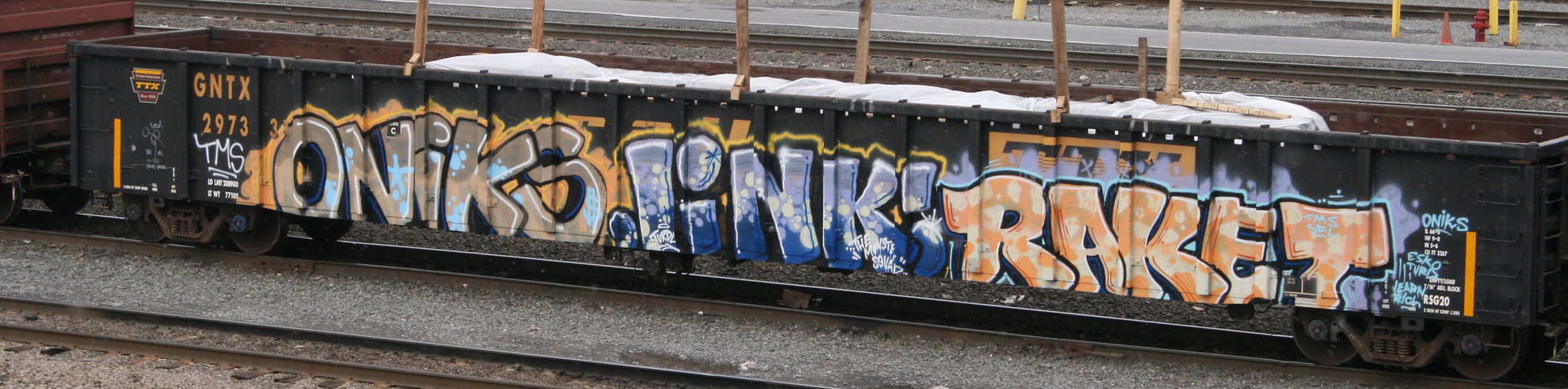The image depicts a long, black metal railroad car attached to a train, approximately 20 to 30 feet in length. The car sits on steel rails, with additional tracks visible in the foreground. The graffiti art on the side of the car features various tags in shades of gray, orange, yellow, tan, and blue. Notably, "ONIKO" or possibly "ONIKO," and "LYNX" are painted in blue, while "RAKET" is rendered in orange. The interior of the car contains some kind of white material secured with straps. Visible on the left side is the marking GN-TX-2973. In the backdrop, there is a concrete subway platform, contributing to the urban setting of the scene.